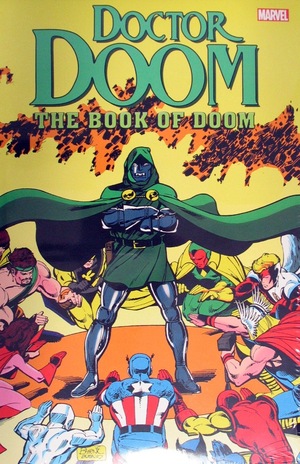This image is a vertically aligned rectangular photo of a comic book cover, with no visible issue number, publisher logo, or price, possibly making it a graphic novel. The top of the cover features large green text with black outlines and drop shadows that reads "Doctor Doom," with "Doctor" in smaller letters than "Doom." Below, in lighter green text with similar black outlines and drop shadows, it says "The Book of Doom." The upper right corner of the cover has "MARVEL" written in all caps with white letters. The background at the top is solid yellow, gradually transitioning to an orange and black splatter pattern.

Taking center stage, Doctor Doom, depicted with a menacing expression, stands with his arms folded over his chest. His face and arms are a bluish hue, and he is clad in a fully metallic suit with a green kilt, hooded cape, and portrayed with two golden pendants at the front. His cape flares out dramatically at the sides. The background behind him features dark, ominous clouds.

Surrounding Doctor Doom are kneeling superheroes from the Avengers, including identifiable characters such as Captain America, Thor, Vision, Iron Man, the Silver Surfer, and Scarlet Witch. These characters bow or kneel toward Doctor Doom on a circular orange floor, their faces and full costumes largely obscured in reverence to the central figure.